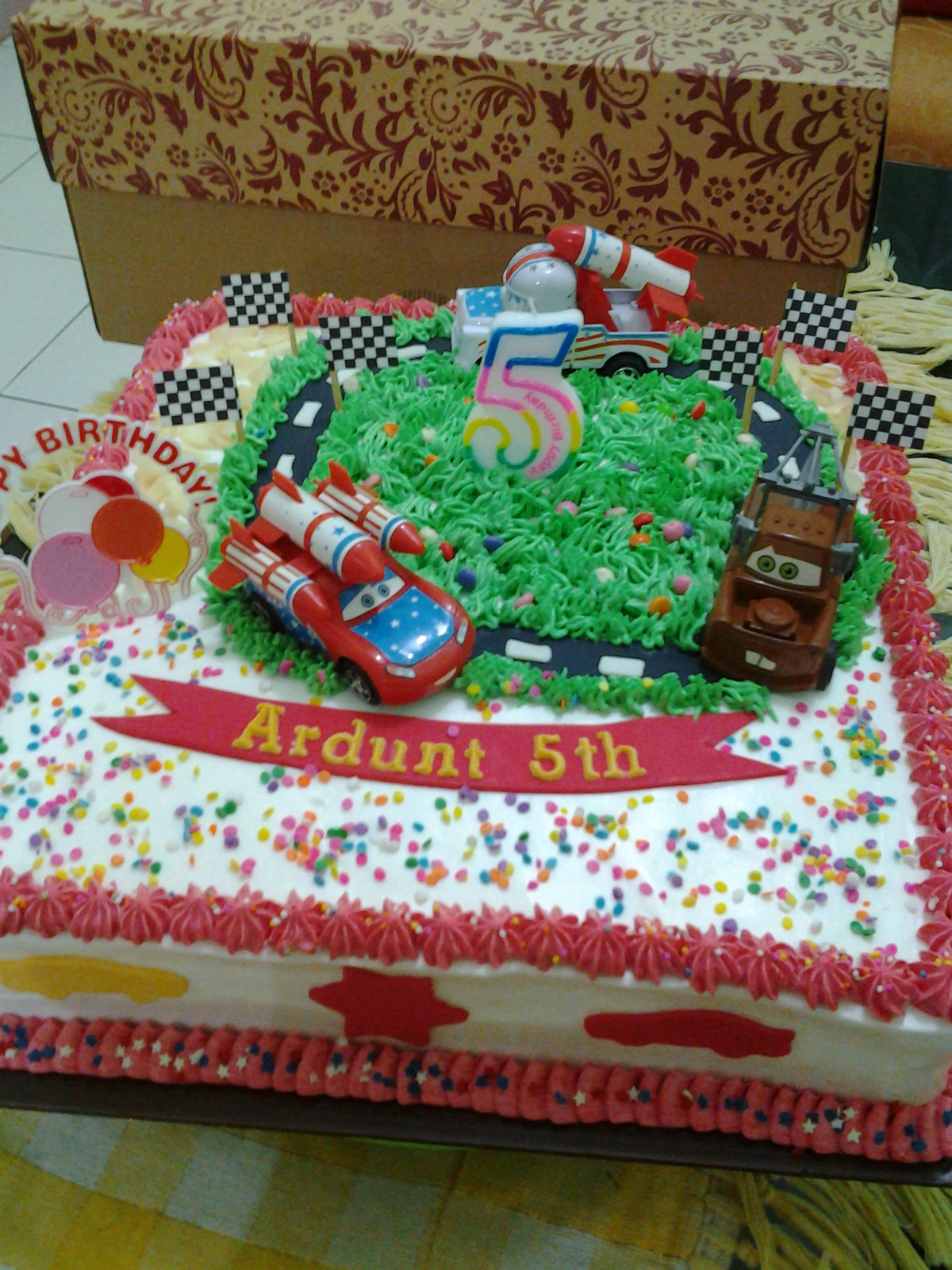In the photograph, we see a rectangular birthday cake designed with a Disney Cars theme, placed on a yellow checkered tablecloth with white tassels at the end. The cake's base is frosted in white and is detailed with red frosting dots along the top and bottom edges. The sides of the cake showcase fondant cutouts, including a red and yellow car, and star shapes. Topping the cake is a red banner that says "Ardent 5th" in gold letters. Scattered across the surface are multi-colored sprinkles resembling confetti.

Central to the decoration is a green icing field representing grass, and there is a dark-frosted racetrack complete with white lines and six checkered flags. On the track are small toy cars, including a red car with a blue hood, adorned with three rockets featuring American flag designs and stars, and a brown tow truck from the Cars movie. A candle shaped like the number five, colored in blue, pink, yellow, and green, sits prominently. Additionally, there are plastic balloon decorations and a "Happy Birthday" sign on the cake, partially obscured so that only the "y" is visible.

In the background, there's a brown box with a floral maroon pattern sitting on a white-tiled countertop, possibly indicating the setting is a kitchen. Elements like a rug and other clear details bring a cozy, homey atmosphere to the image.